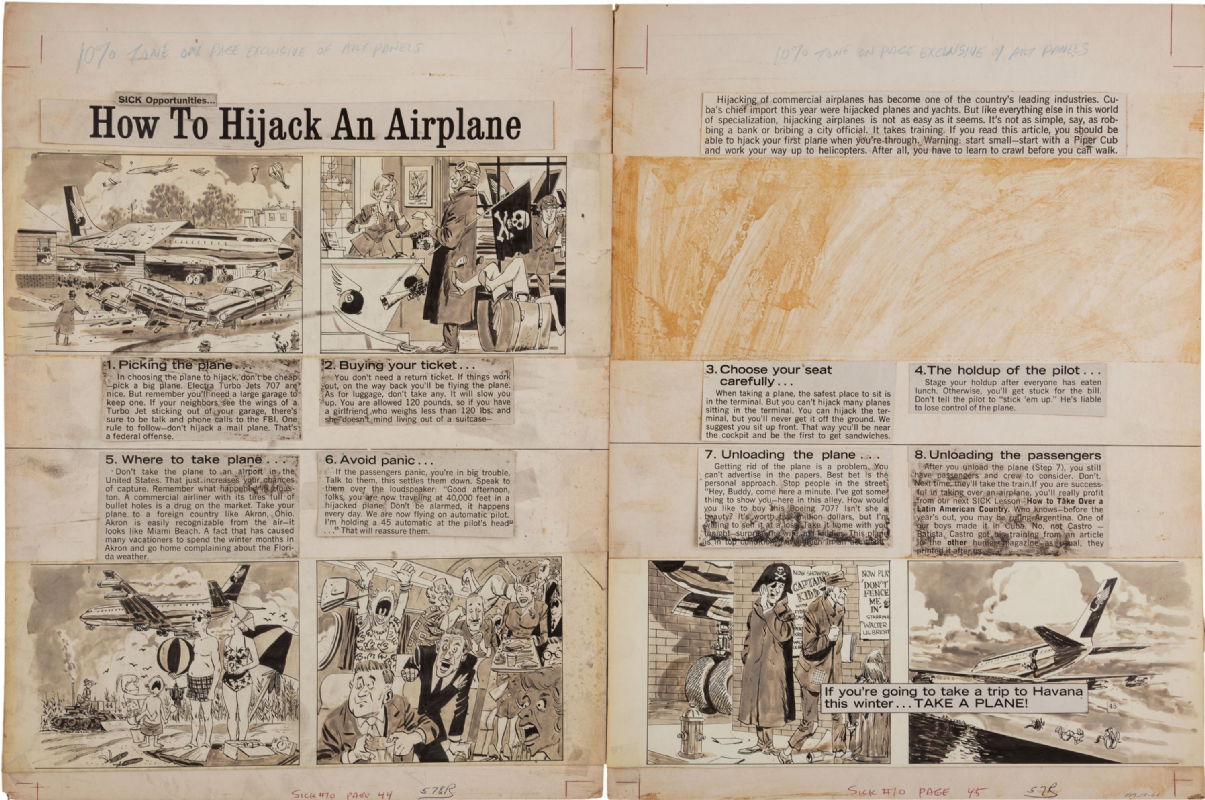The image features a worn and yellowed old magazine or pamphlet opened to two of its interior pages. The title at the top of the left page reads "How to Hijack an Airplane." This section details an eight-step process for hijacking a plane, listed in numerical order: 

1. Pick a plane 
2. Buy your ticket 
3. Choose your seat 
4. Hold up the pilot 
5. Decide where to take the plane 
6. Avoid panic 
7. Unload the plane 
8. Unload the passengers

The pages include various comic-style illustrations depicting scenes from the hijack experience, such as an airplane in a hangar, people inside an airport with a pirate flag, terrified passengers, and a man with a gun holding up someone at the airport. The paper quality reflects its age, with visible deterioration, yellowing, and some stains. There are also additional cartoon panels and explanatory text, suggesting a step-by-step visual guide. At the bottom of the section, there is a note about taking a trip to Havana in winter, adding an oddly specific travel detail to the otherwise sinister content.